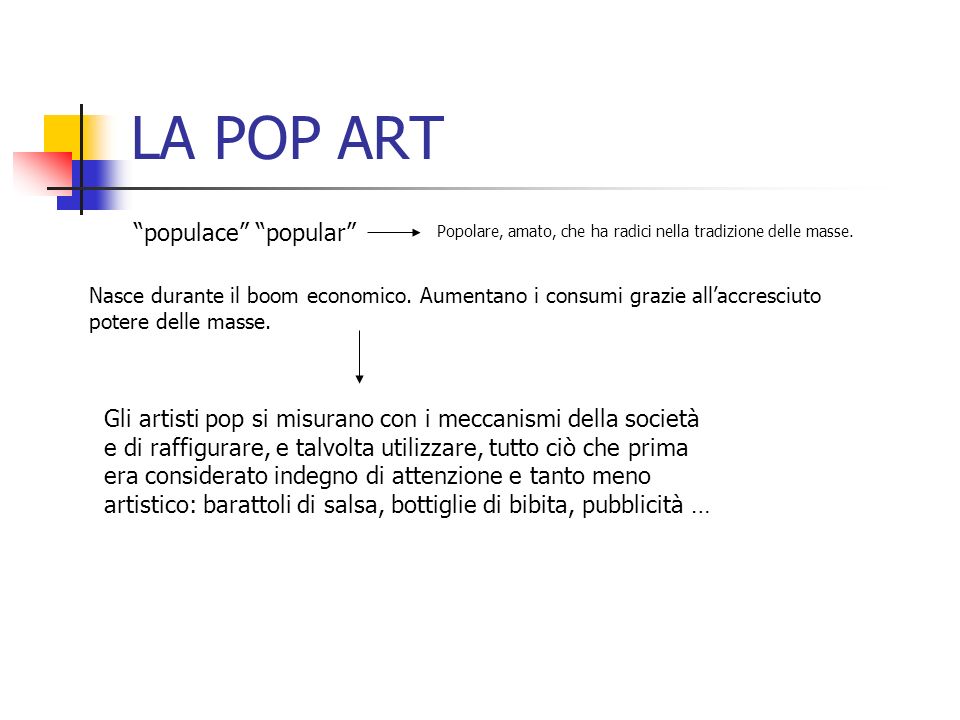The slide, possibly from a presentation, prominently features the title "LA Pop Art" in navy blue, all-caps lettering at the top. To the left, there is a logo consisting of three squares: a pinkish-red square on top, a yellow square in the middle, and a blue square on the bottom, each one fading outward. Below the title, a horizontal line fades off to the right, creating a separator from the text below. 

The heading beneath the line includes "Populus" and "Popular" in quotes, followed by an arrow pointing right to a series of Italian words: "Populare, Amato, Sheha, Radici, Nella, Tradizioni, Della, Masse." Larger text below this reads: "Nasse Durante Il Boom Economico, Amentano I Consumi, Grazie Al Acresucito Potere Delle Masse." Another arrow points downward to slightly larger text, which describes in Italian how pop artists engage with societal mechanisms, emphasizing the artistic transformation of mundane items, such as soup cans and beverage bottles. The text highlights how these artists reframe what was once deemed unworthy of attention, with a concluding ellipsis (...). All text appears in a simple black font, specifically Alba.